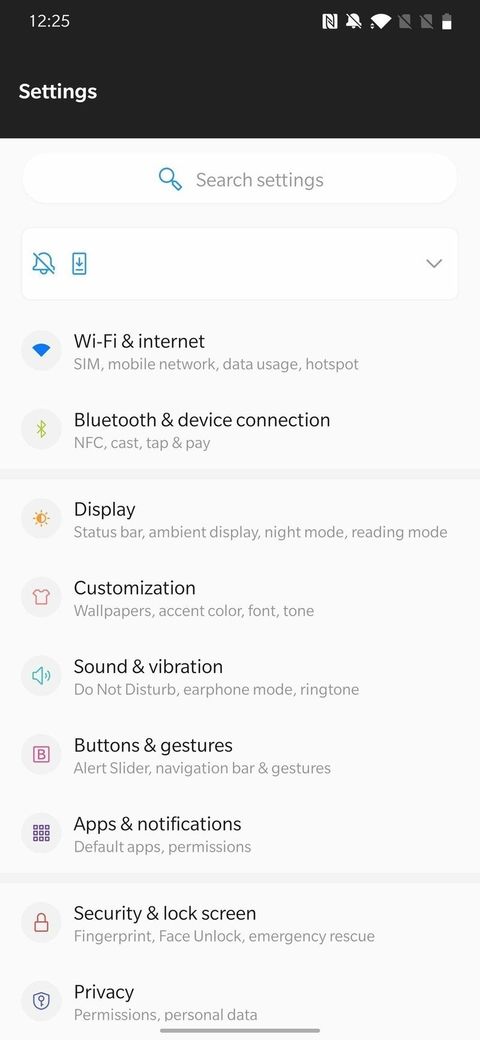This image depicts the settings section of a device interface, presented on a black background. At the top left corner, the time is displayed as 12:25, accompanied by a bold "Settings" title. The top right corner features a series of small icons, although their details are obscured by the image's size. 

The first line of the interface presents a "Search settings" field within a white box, including a magnifying glass icon. Below this, there is a bell icon with a line through it, followed by what appears to be a battery icon.

The main settings categories are listed below these icons, each accompanied by relevant sub-options and icons to their left:

1. **Wi-Fi & Internet**: 
    - Sub-options: SIM, Mobile Network, Data Usage, Hotspot.

2. **Bluetooth & Device Connection**: 
    - Sub-options: NFC, CAST, Tap & Pay.

3. **Display**: 
    - Sub-options: Status Bar, Ambient Display, Night Mode, Reading Mode.

4. **Customization**: 
    - Sub-options: Wallpapers, Accent Colors, Font, Tone.

5. **Sound & Vibration**: 
    - Sub-options: Do Not Disturb, Earphone Mode, Ringtone.

6. **Buttons & Gestures**: 
    - Sub-options: Alert Slider, Navigation Bar and Gestures.

7. **Apps & Notifications**: 
    - Sub-options: Default Apps, Permissions.

8. **Security & Lock Screen**: 
    - Sub-options: Fingerprint, Face Unlock, Emergency Rescue.

9. **Privacy**: 
    - Sub-options: Permissions, Personal Data.